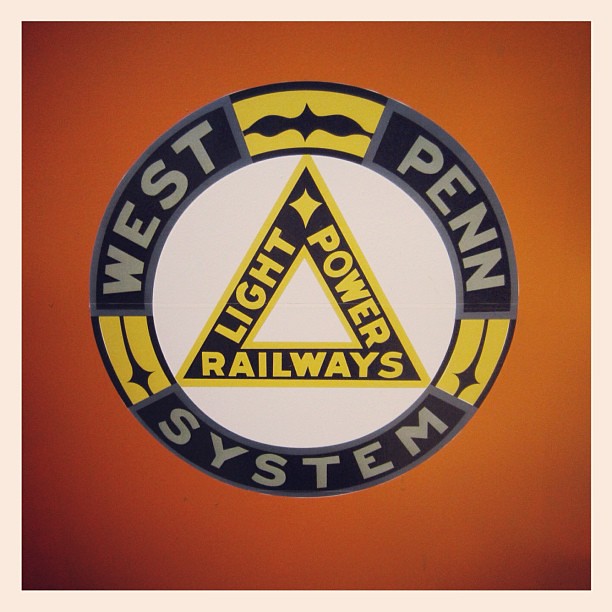The image features a vintage-style logo against a gradient burnt orange background, transitioning from light orange at the center to black or dark burnt orange at the corners. Encasing the entire image is a peach-colored border, creating a framing effect. Central to the logo is a circular design, outlined with a gray line and an alternating thin border of yellow and black segments. Within this circle is another white circle containing a yellow-bordered triangle with a black banner inside. The banner displays the words "LIGHT" on the left, "POWER" on the right, and "RAILWAYS" at the bottom, all in yellow capital letters. Additionally, around the perimeter of the circle, the text reads "West Penn System," with "WEST" to the left, "PENN" to the right, and "SYSTEM" at the bottom, separated by yellow segments. The overall aesthetic suggests that this logo is for the West Penn System Light Power Railways, characterized by its old-fashioned, nostalgic design.